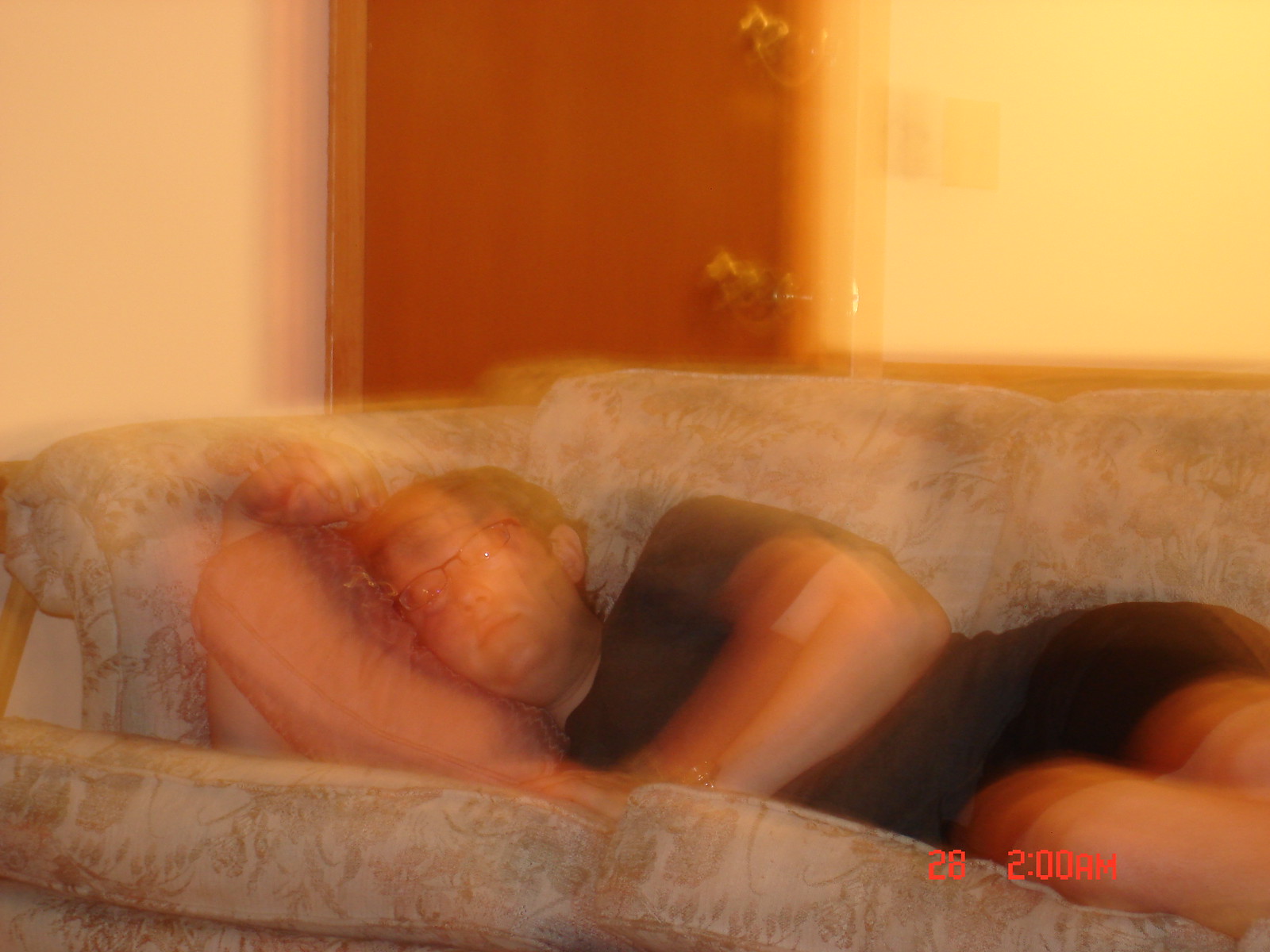This indoor photograph, characterized by its blurry, double-exposed quality, captures a man wearing glasses, a black short-sleeved shirt, and black shorts, reclining on a flower-patterned couch. He is lying on his right side with one arm behind a pillow that supports his head and the other arm resting in front of him. The couch features a beige color with floral designs. The background reveals an off-white or white wall and a wooden door with a bronze door handle, a deadbolt lock, and a light switch to its right. There’s a time stamp in the bottom right-hand corner that reads "28-2AM" in red.